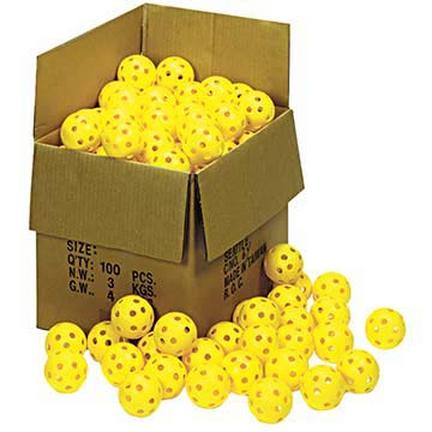The photograph features a brown cardboard box overflowing with plastic yellow balls, identifiable as either wiffle balls or pickleballs. The box is placed against a solid white background, creating the illusion that the objects are floating. The front flaps of the box are folded downwards, while the back flaps are pointing upwards. A multitude of black text printed on the sides of the box includes: "size," "quantity 100 pieces," "NW 3 KGS," and "GW 4." However, sections of the text are illegible, and one side possibly indicates "Made in Taiwan." Each round ball is perforated with multiple holes, some of which are visible through to the other side. The abundance of yellow balls fills the box beyond capacity, with additional balls scattered in front of it, enhancing the sense of overflow.